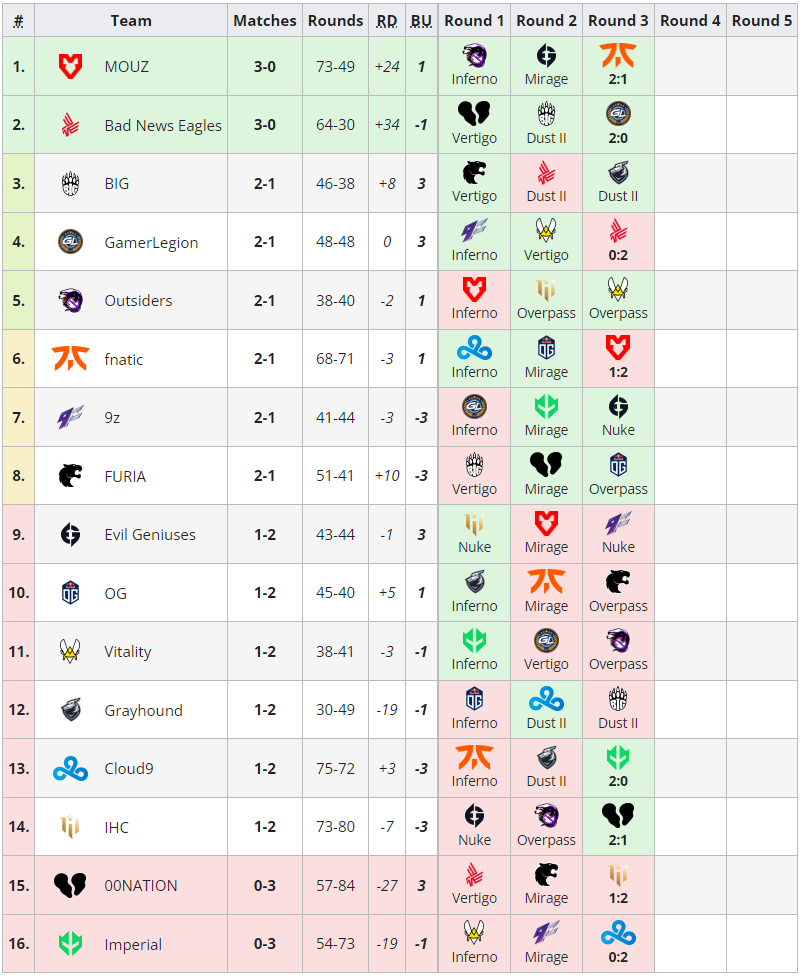This image is a screenshot of a detailed gaming league competition spreadsheet. The spreadsheet is organized meticulously, featuring a menu bar across the top with gray boxes highlighting various categories. These categories include: Ranking Number, Team, Matches, Rounds, RD, BU, followed by Round One through Round Five. Completion data is noted only for Rounds One through Three.

Vertically along the left side, the ranking numbers are listed from 1 to 16, accompanied by each team’s logo for easy identification. The match wins for each team are prominently displayed in bold black text. Notably, the top two teams are highlighted with light blue boxes, while the bottom two teams are marked with pink boxes. The spreadsheet uses color coding to indicate match outcomes, with blue denoting a win and red indicating a loss, thereby displaying the results of the matches each team has participated in.

This well-structured and visually clear layout makes the document easy to read and understand, suggesting it is designed to track and present the standings within a gaming competition.